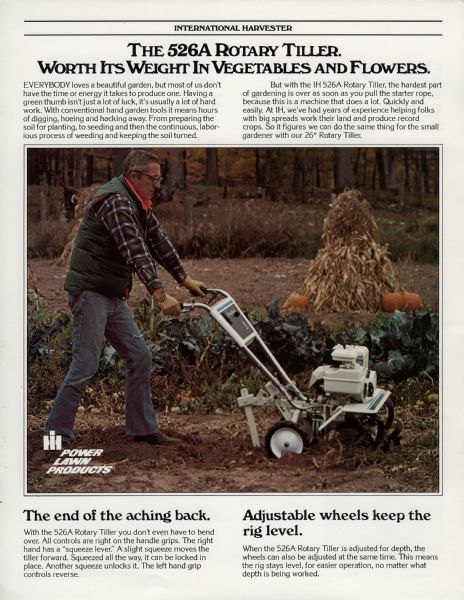This vertical image appears to be a page from an older magazine or newspaper, featuring an advertisement for the International Harvester 526A Rotary Tiller. The beige paper includes a black-inked title at the top, flanked by two horizontal bars, reading "International Harvester, the 526A Rotary Tiller, worth its weight in vegetables and flowers." The body of the text explains how the 526A Rotary Tiller simplifies gardening, making the hardest parts of the process—such as digging, hoeing, and weeding—effortless by merely pulling the starter rope. The article also notes that adjustable wheels on the tiller keep the rig level, preventing back strain.

Dominating the center of the page is a square-shaped image of a white man, in his 30s or 40s, with short gray hair and glasses. He is dressed in jeans, a green vest, a red, white, and blue plaid shirt, and tan gloves. The man is operating the white rotary tiller, which features wheels, an engine, and a handle, tilling a field of dirt and vegetables. Two smaller captions accompany this picture: "Power Lawn Products" in white text on the bottom left, and "The end of the aching back; adjustable wheels keep the rig level," in black ink at the bottom.